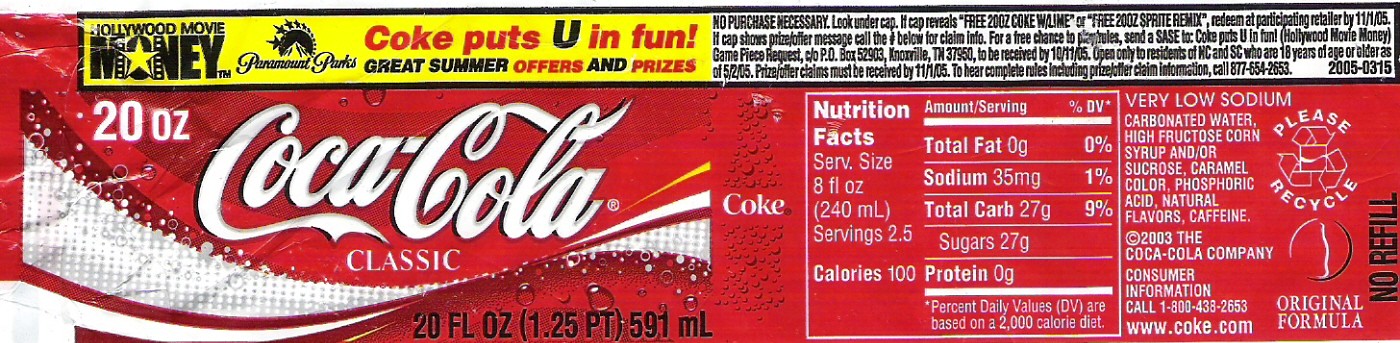This image captures a laid-out Coca-Cola bottle label on a flat surface. The dominant color of the label is a vibrant red, accented with white text and additional design elements. On the left side, the main label section prominently displays the Coca-Cola Classic logo, accompanied by a white ribbon design at the bottom. Above this logo, to the top left, the label indicates the bottle size as "20 ounces," repeated below in finer details as "20 fluid ounces (1.25 pint / 591 ml)." 

Centered on the label's top section, there is a black-outlined rectangular box with a yellow banner on the right. This section features several promotional texts, including "Hollywood Movie Money" alongside the Paramount Pictures logo. The text "Coke Puts You in Fun!" is highlighted in red, and an additional promotional phrase reads "Great Summer Offers and Prizes."

To the right of the main label, the right side of the image contains detailed nutritional information and ingredients listed in white text. The nutrition facts table includes values for total fat, sodium, total carbohydrate, sugars, and protein. Below this table, a recycling symbol is visible, reinforcing the brand's environmentally conscious messaging.

Overall, the label melds branding, bottle-specific details, promotional offers, and essential consumer information in a cohesive and eye-catching design.